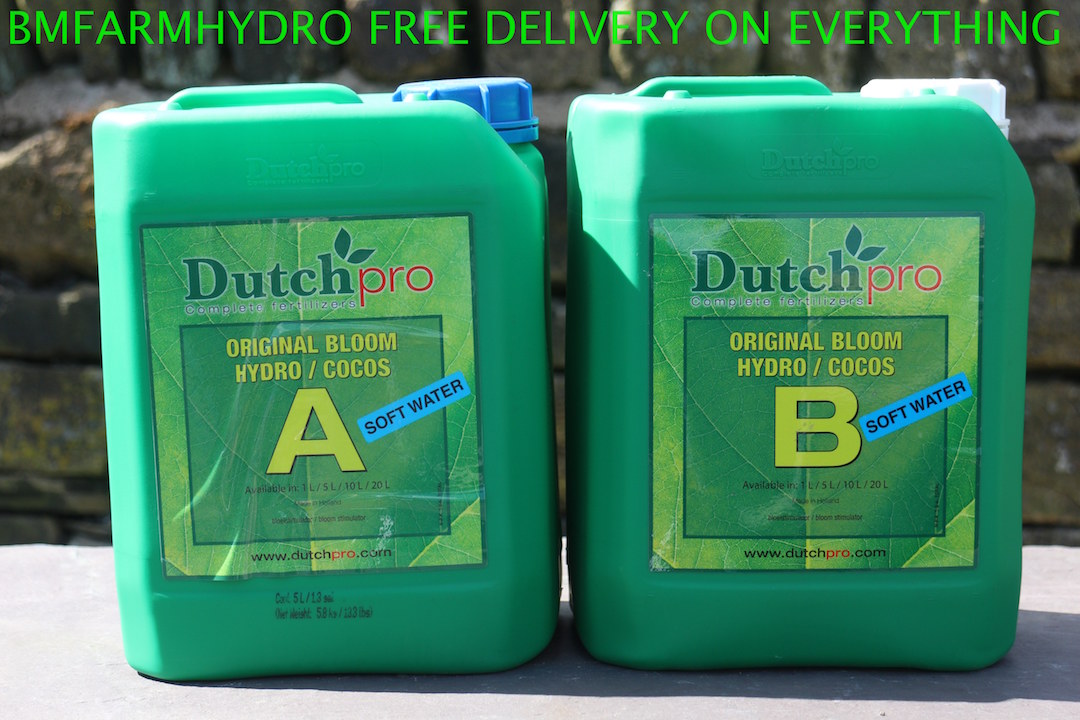The image is a close-up shot of two green plastic containers, likely jugs, of Dutch Pro Original Bloom Hydro/Cocos, an agricultural product. The container on the left features a blue cap and a label that reads "Original Bloom Hydro/Cocos A", with a prominent yellow 'A' and a blue label indicating "soft water". The container on the right has a white cap and bears the label "Original Bloom Hydro/Cocos B", with a prominent yellow 'B' and the same blue "soft water" label. Both containers have the Dutch Pro brand name in green text. They are positioned on a gray stone surface with a stone wall in the background, suggesting the photo was taken outdoors on a sunny day. Overlaid at the top in green text are the words "BM Farm Hydro free delivery on everything".